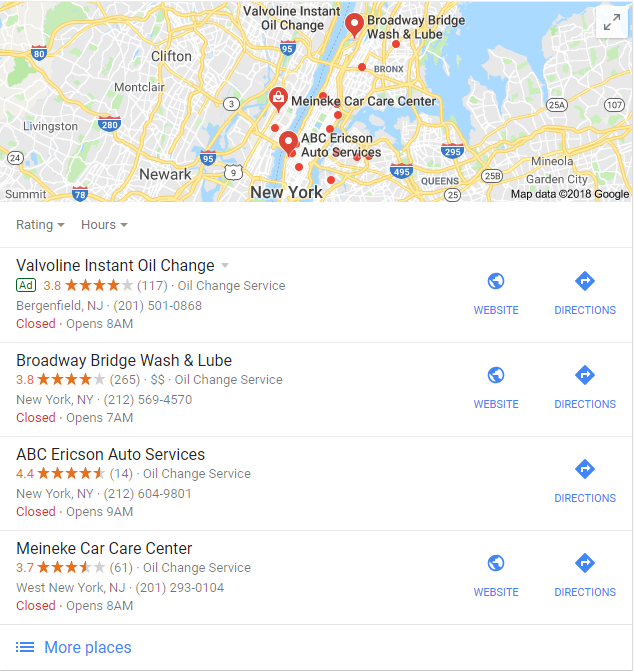The image resembles a Google Maps interface, depicting a map of a region with "New York" labeled in black text at the bottom. Scattered across the map are numerous small red dots and more prominent red markers indicating various locations. The map also features names of different places in black text, such as "Valvoline Instant Oil Change," "Broadway Bridge Wash and Lube," "Clifton," "Newark," and "Livingston." Yellow roads are visible crisscrossing the area, along with blue regions, presumably bodies of water.

Below the map, there is a list of places. At the top of the list is "Valvoline Instant Oil Change," accompanied by a rating of 3.8 stars, described as an oil change service that is currently closed but opens at 8 a.m. Links for the website and directions are provided to the right. Following this are several other listings: "Broadway Bridge Wash and Lube," "ABC Erickson Auto Services," and "Meineke Car Care Center." All these entries have ratings, indicate they are oil change services, and note that they are currently closed.